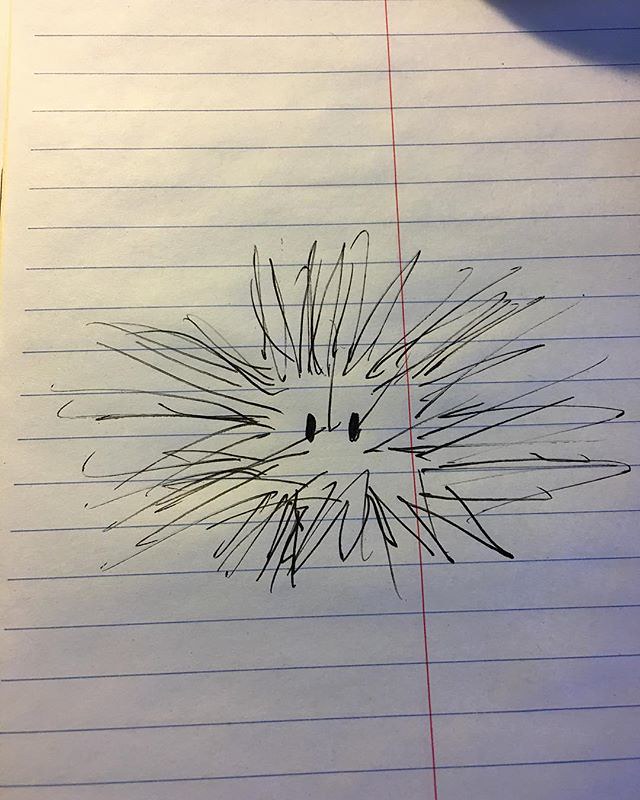The image depicts a piece of white notebook paper with horizontal blue lines and a vertical red margin line running down the center of the page. In the middle of the page, there is a whimsical drawing made with either a black ink pen or a fine-point black marker. The drawing features two vertically oriented, black-filled oval eyes positioned within an implied, but not explicitly drawn, circular form. Surrounding the eyes and the central space are numerous jagged, scratch-like lines and V-shaped marks, creating the appearance of a spiky, hairy creature. The markings extend outward, giving the figure a chaotic, scribbled texture. In the upper right corner of the paper, a shadow is present, casting a subtle darkness. Additionally, part of a blue object and a beige surface, likely a desk, are visible in the photograph, suggesting the notebook is resting on it.